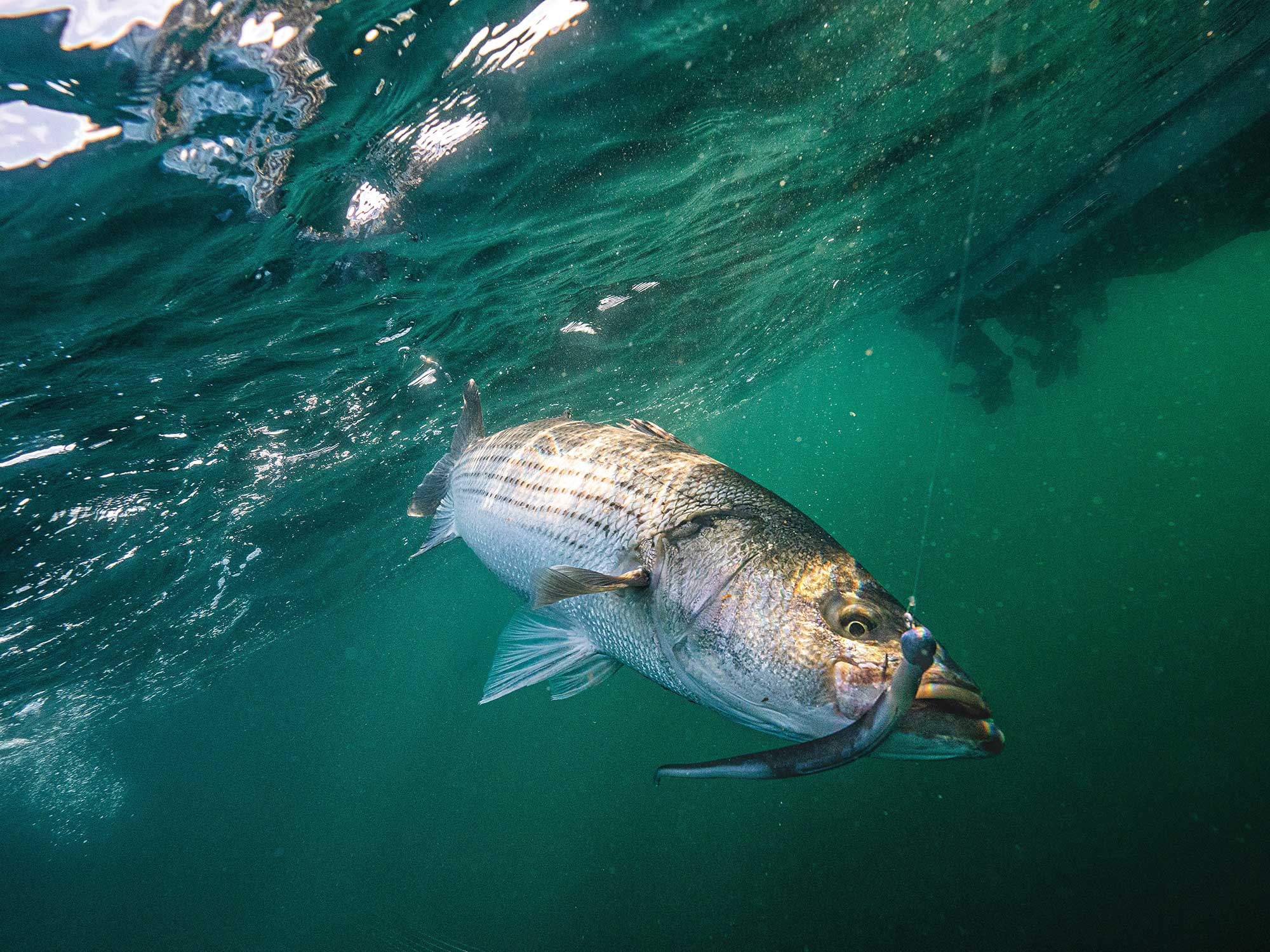The photograph captures a striking underwater scene of a large fish in crisp focus, moments away from a fishing lure. The fish is centrally positioned, its body slightly below the water's surface, with sunlight filtering down from above, illuminating its black-scaled back and white underbelly. The fish appears long and robust, featuring prominently large lips and an underbite. A metal hook with a realistic, fish-shaped lure dangles tantalizingly in front of its mouth, the hook visibly piercing its lip in painful detail. The water is clear with a greenish hue, and the surface is slightly tilted counterclockwise. Bubbles and minor disturbances in the water can be seen, suggesting recent activity, possibly from the fish breaching and re-entering the water. Adding depth to the scene, the silhouette of a boat with propellers is faintly visible in the upper right corner, indicating the presence of fishermen above. The entire composition offers a dramatic snapshot of the underwater battle between fish and fisherman, set against a backdrop of natural light and fluid dynamics.